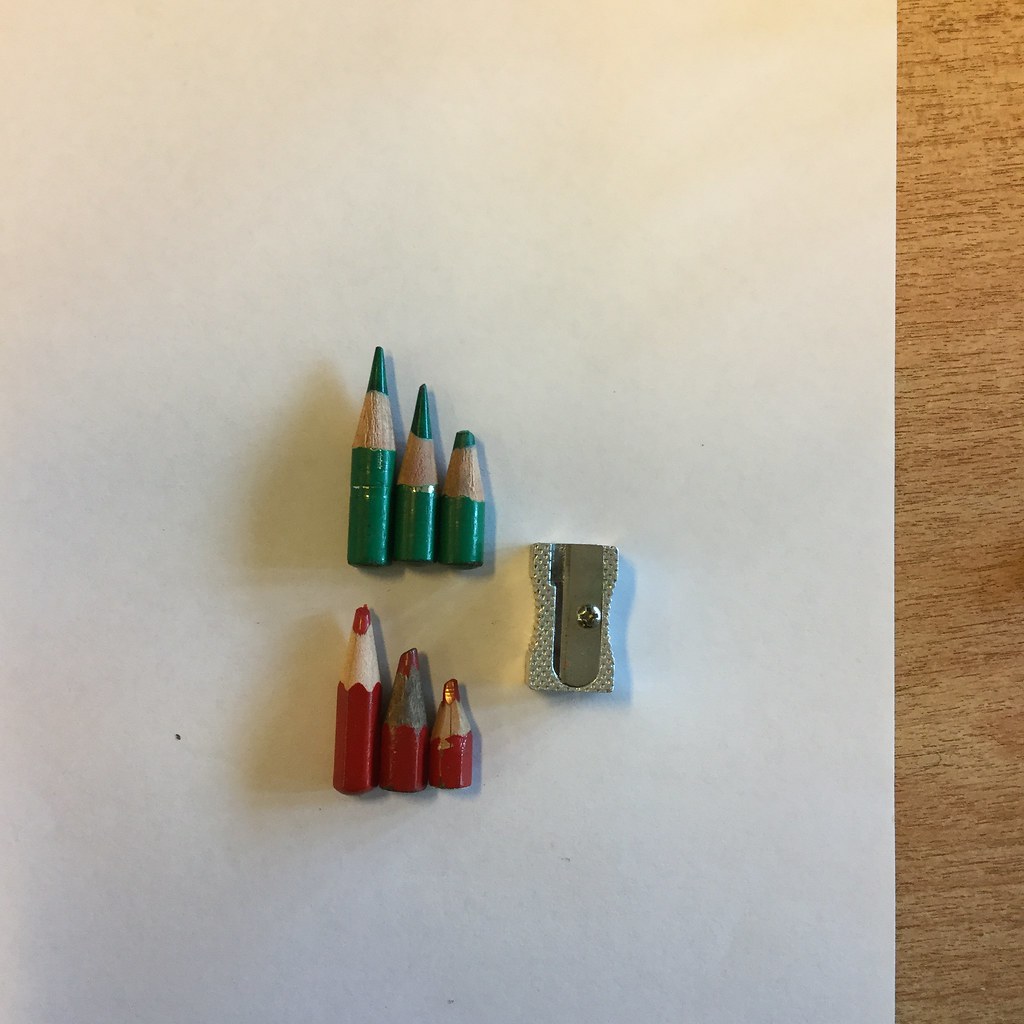This photograph features six dramatically shortened colored pencils displayed on a piece of white paper laid over an orange wooden surface with a fine grain. The pencils, which consist of three green ones on top and three red ones on the bottom, are arranged in descending order from left to right, with the tallest on the left and the shortest on the right. Due to excessive sharpening, the pencils appear dented and damaged along their sides, with each resembling minuscule stubs barely reaching an inch in height. A stainless steel pencil sharpener with a textured grip for ease of use is situated to the right of the pencils, slightly shorter than the tallest pencil. Soft shadows cast by the pencils indicate a light source from the right, adding depth to the composition.